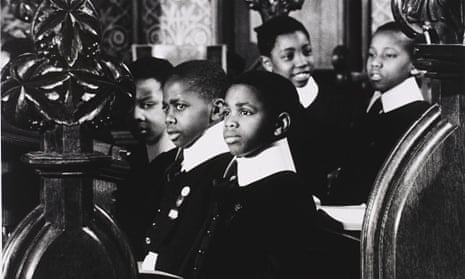In this black and white photograph, five young black boys, likely members of a church choir, are seated in ornately carved wooden pews. They are dressed in black uniforms adorned with large, high white collars and ornate buttons. One boy in the front has a medal pinned to his coat, suggesting an award or form of recognition. The three boys in the front, appearing to be around seven to eleven years old, have short black hair and wear serious expressions as they look off to the left. Behind them, two other boys—one facing forward with a smile, the other looking at him—seem to be in a lighthearted conversation. The wooden pews they're seated in feature intricate carvings, adding to the church-like atmosphere suggested by the walls in the background. The overall scene emanates a historical and solemn ambiance, reflective of a formal church setting.